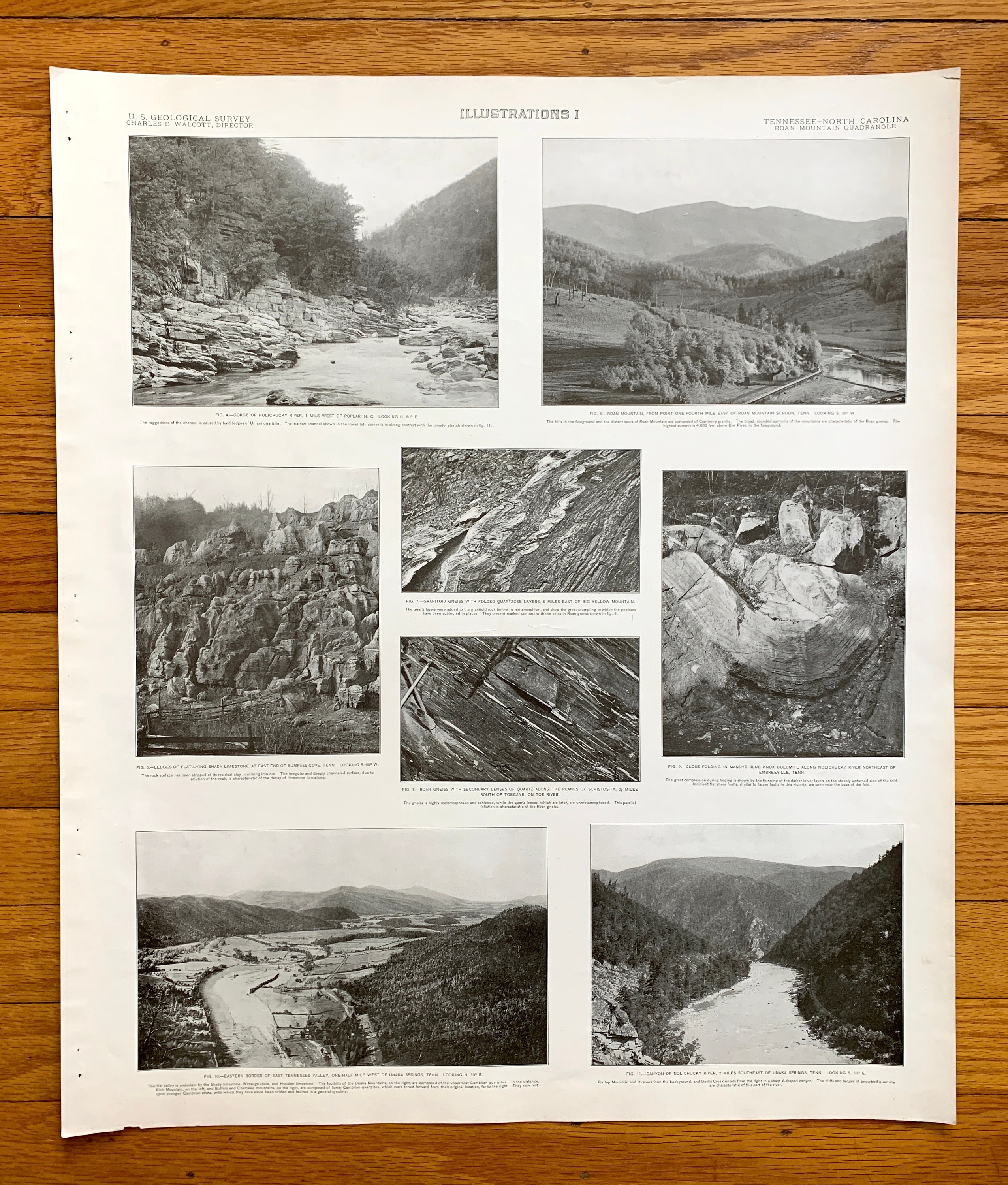The photograph depicts a slightly aged off-white page from an illustrations book, labeled at the top with "Illustrations 1" and flanked by the "U.S. Geological Survey" on the upper left, specifying Charles D. Walcott as the director. On the upper right, it notes "Tennessee, North Carolina Roan Mountains quadrangle." The page displays a collage of eight black and white photographs against a white background. The upper row features two side-by-side photos: to the left, a stream meandering through a rocky, cliff-like terrain with overhanging trees; to the right, an aerial view of a misty mountain surrounded by flatlands and dense forest. The middle section consists of four photographs showcasing various rock formations and weathered stone cuts. The bottom row includes two photographs: on the left, a valley with winding water, and on the right, a stream flowing through a hilly area with a waterfall and distant mountains. The page lies on a yellowish, golden brown wooden surface.